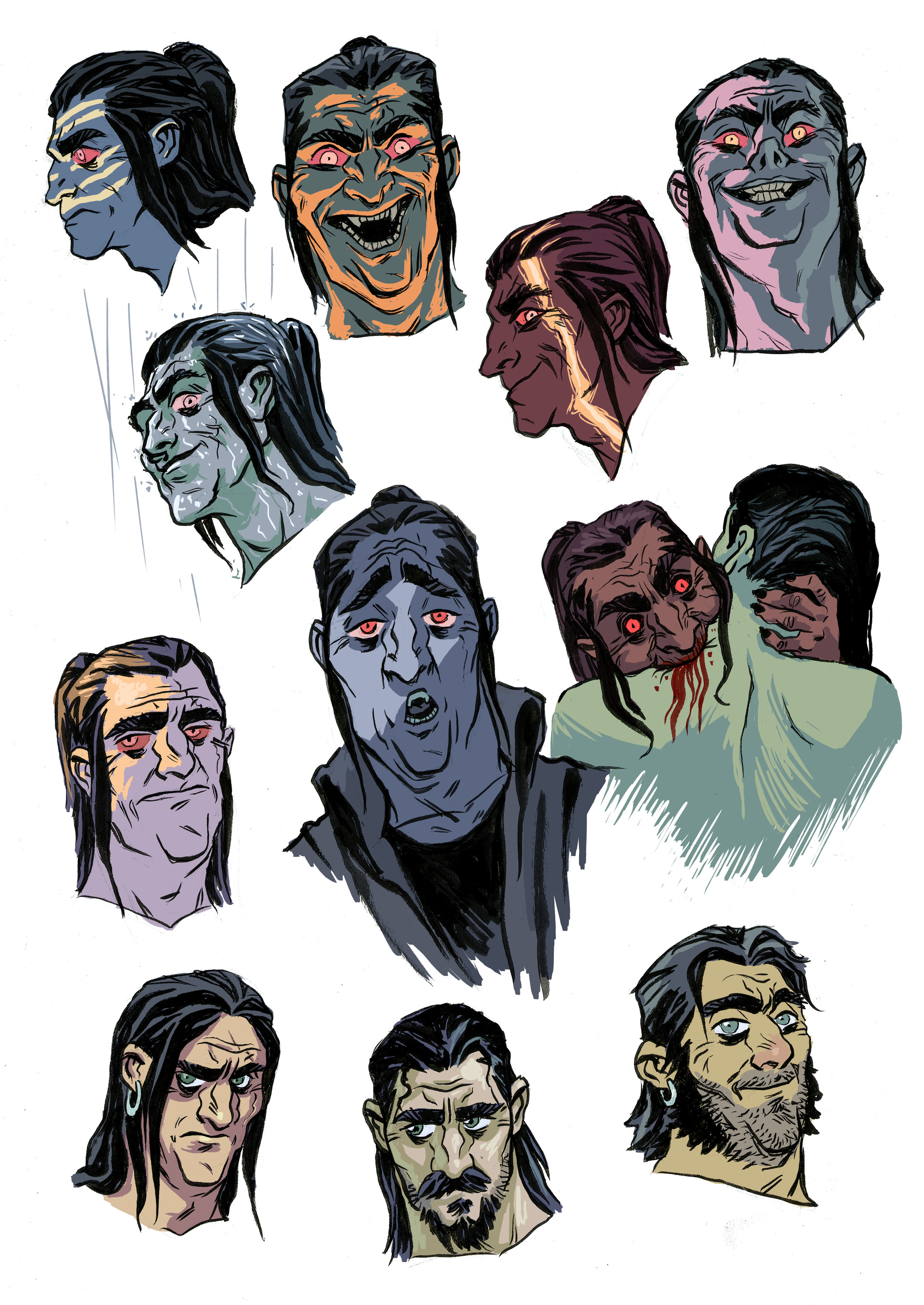The illustration presents a series of detailed images depicting various angles and personalities of a single male character who transforms between vampire and human states. Central to the composition is a menacing vampire with long dark hair tied up in a ronin-style bun, characterized by his red eyes and pointy fangs. His dark grey skin and shadowy appearance add to the sinister aura, particularly in the image where he opens his mouth wide, revealing his sharp teeth while looking towards the viewer. 

In several top images, the vampire’s face alternates between bluish, yellowish, and purple hues, showcasing his different expressions such as a sinister grin and a ferocious snarl. One notable scene captures him in the act of biting a woman's neck, with blood vividly protruding from his mouth and her shoulder, accentuating his predatory nature.

Towards the bottom of the illustration, the character appears more human with a normal skin tone, a black moustache, and beard, and blue eyes, which starkly contrast the previous red-eyed, vampiric depictions. Here, the character’s expressions are more relaxed and content, with light cascading across his face, giving a softer, more approachable appearance compared to the top images beset by deep shadows. This transformation from a dark, shadowy figure to a more light-infused human-like portrayal underscores the multifaceted nature of the character.